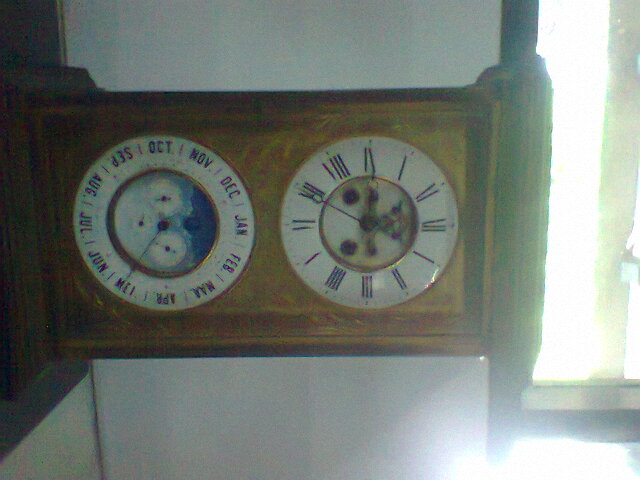This photograph captures a uniquely oriented wooden clock with a calendar dial, set against the backdrop of a bright white indoor wall. The clock, which appears old with visible scratches and fading, is positioned horizontally across the frame, presenting an unusual yet intriguing layout. The left side of the clock features a calendar dial with the months of the year displayed around its border in clockwise fashion, highlighted by a blue inner circle adorned with a cloudy sky design and pointers indicating the current month. Nested within this calendar dial, there are three smaller mysterious dials whose functions are unclear. On the right-hand side of the clock, a traditional clock face showcases Roman numerals and red clock hands, with a partial view of its internal gears visible. Adjacent to the clock, to the far right of the image, a window bordered by dark brown wood allows bright sunlight to illuminate the indoor setting, creating a stark contrast with the soft natural lighting. The picture also provides a glimpse of a brown-shaded floor on the left and a light brown wooden surface enhancing the overall warm aesthetic against the picture’s broader square frame.